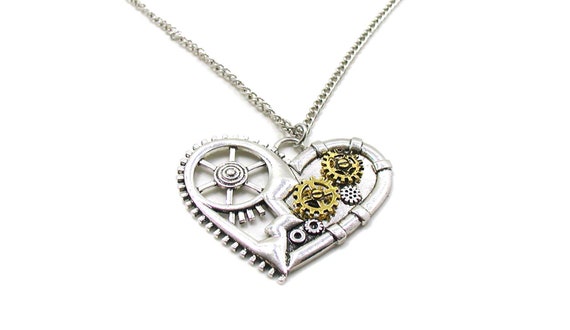The image features a steampunk-style necklace with a distinctive heart shape, predominantly silver in color. This heart-shaped pendant is intricately composed of several gears and cogs, highlighting an industrial aesthetic. The left half of the heart showcases a smooth silver outline, with a broken heart design down the center and a chain-like effect along its edge containing a prominent silver gear. The right half of the heart is embedded with five gears varying in size; two are larger and brass or copper-colored, while the remaining three are smaller and golden. Small circles accentuate the bottom of the heart, adding to its complex design. The pendant is paired with a thin silver chain, suitable for wearing around the neck. The entire piece is set against a white background typical of product page displays, emphasizing its potential as a purchasable item or printable image.